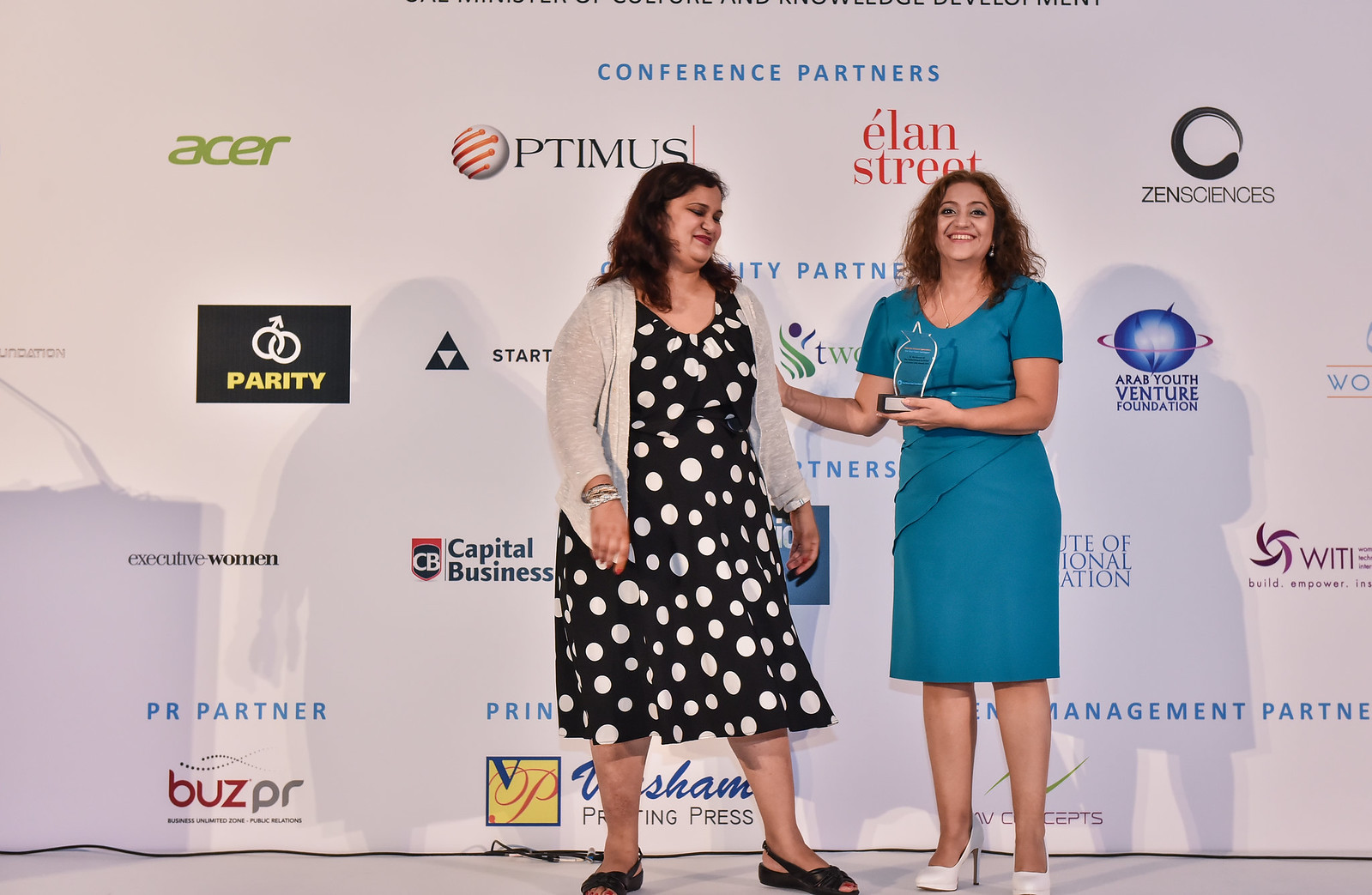In this detailed photograph taken at a conference, two women are standing side by side on a stage against a white background adorned with various sponsor logos, including Acer, Elan Street, Zen Sciences, Arab Youth Venture Foundation, Capital Business, PR Partner, and more. The woman on the right, with brown curly hair cascading down the sides of her face and covering her ears, is beaming a wide smile that shows her top row of teeth. She is dressed in a light blue knee-length skirt suit with sleeves just below her shoulders and white high-heeled shoes. In her left hand, she holds a plaque-like award with a glass top, extending it towards the other woman, her right hand gently resting on her companion's arm.

The woman on the left, slightly overweight with long brown hair, shyly looks down at the award with a humble smile, her eyes closed. She is attired in a black dress with white polka dots, over which she has draped a tan sweater, and she is wearing black sandals. Both women cast shadows on the wall behind them, adding depth to the image. The scene encapsulates a moment of recognition and appreciation, highlighting the joyful expression of the presenter and the modest demeanor of the recipient.